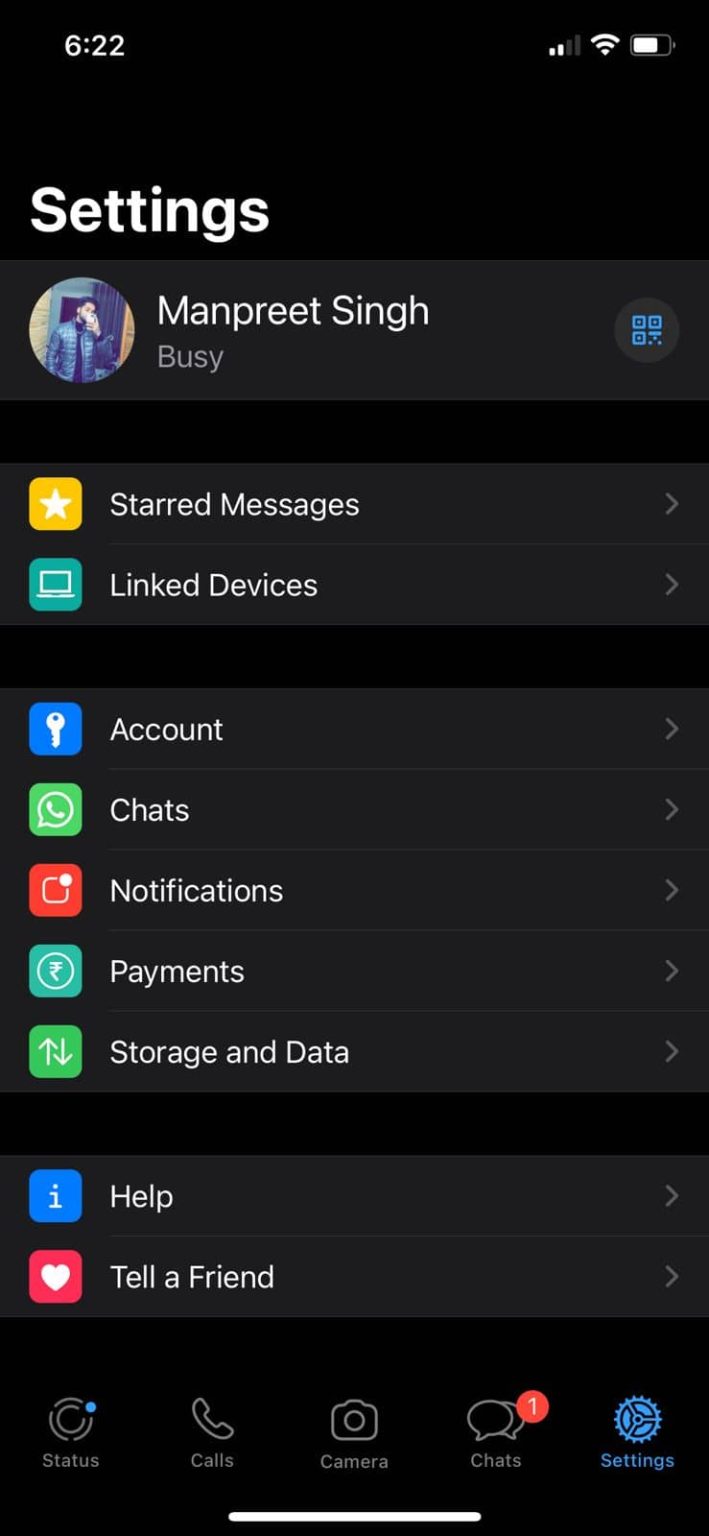The image is a screenshot of the settings section on a smartphone. At the top left corner, the time is displayed as 6:22. On the right side of the top bar, there are several icons in sequence: a data (network) icon, a WiFi icon, and a battery icon. Below the top bar, on the left side, the word "Settings" is prominently displayed. Adjacent to this is a profile picture of an individual taking a photo in a mirror, labelled with the name "Manpreet Singh" and the status "busy." The main section of the screenshot shows a list of different settings categories, including "Starred Messages," "Linked Devices," "Account," "Chats," "Notifications," "Payments," "Storage and Data," "Help," and "Tell a Friend."